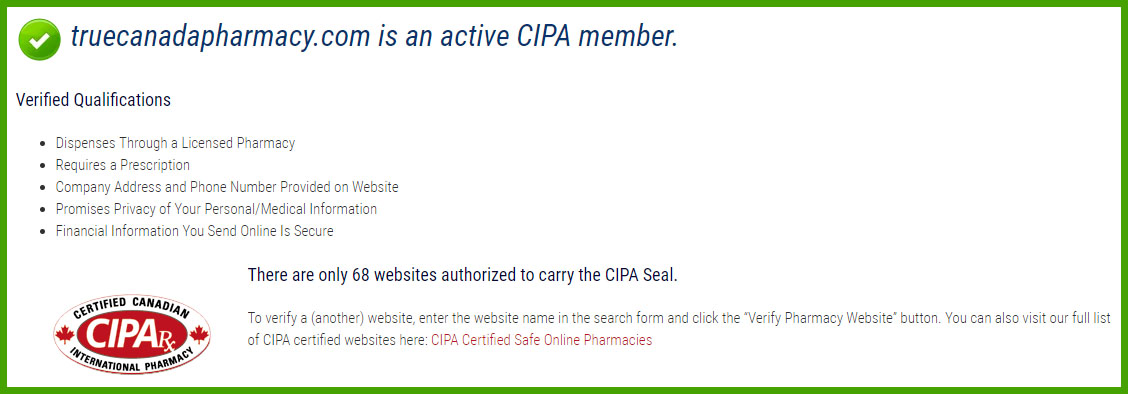The image is a detailed screenshot of an informational box from a website. In the top-left corner, there is a green square with a white check mark inside it, indicating a positive status. Below the square, in bold text, it reads, "truecanadapharmacy.com is an active CIPA member." Following this declaration, there are several bullet points that highlight the pharmacy's credentials and security measures, including:

- Dispenses through a licensed pharmacy.
- Requires a prescription.
- Company address and phone number provided on the website.
- Promises privacy of your personal/medical information.
- Ensures the financial information you send online is secure.

In the middle of the information box, additional context is provided, stating, "There are only 68 websites authorized to carry the CIPA seal. To verify another website, enter the website name in the search form and click the verify pharmacy website button." Furthermore, the text encourages users to "also visit our list of CIPA certified websites here," with a clickable link provided for convenience.